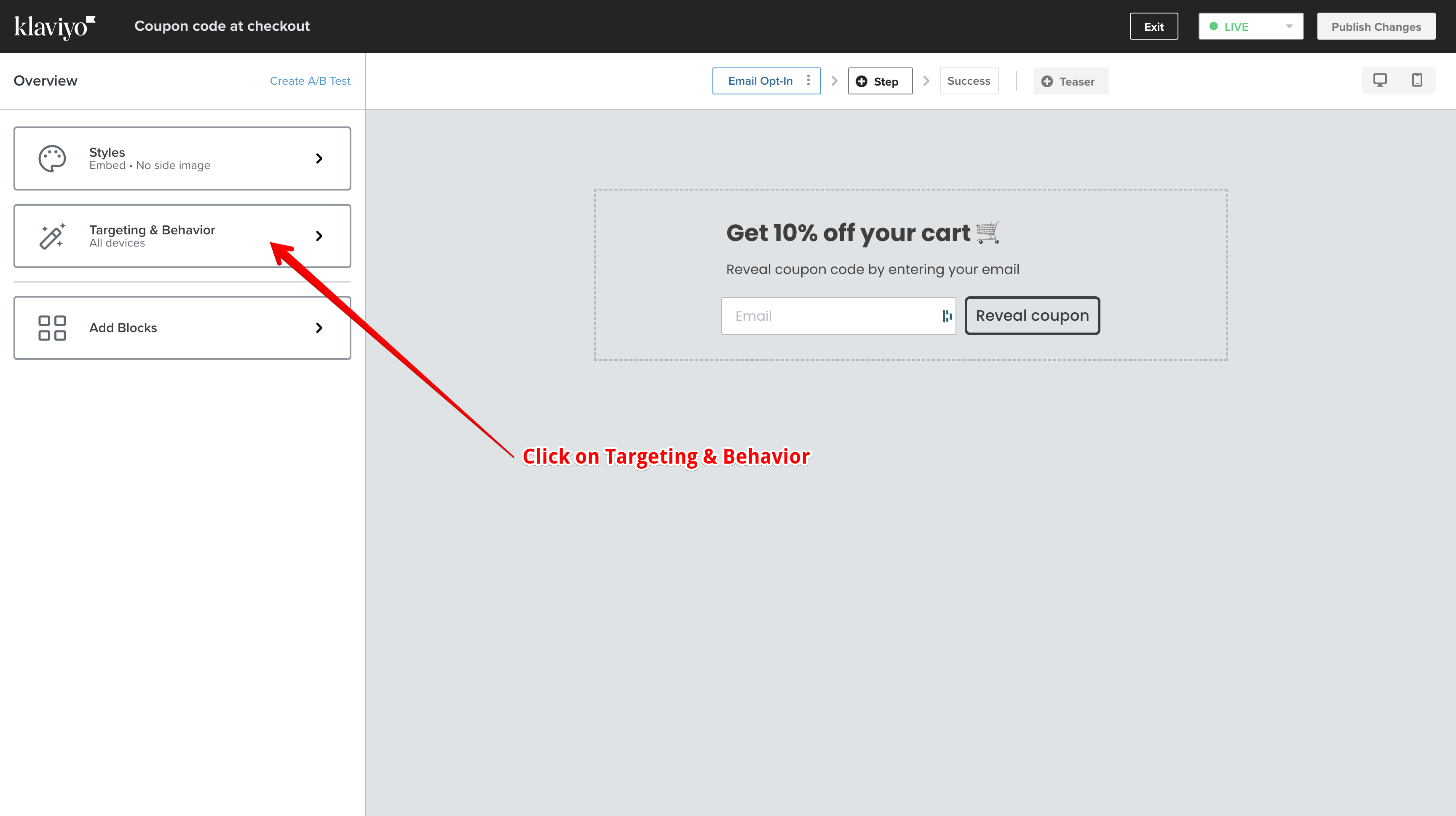The image features a user interface for an online promotional platform. At the top, there's a black header with the text "KLAVIO" in white on the upper left, followed by "Coupon code at checkout" also in white. Below this header, in the middle, there are several interactive elements. 

Starting from the left, a small white box with the word "Exit" is visible. Adjacent to it, a green box with a green circle contains the label "Live." To the right, there is a gray box with darker gray text that reads "Publish Changes." 

On the left side of the interface, the word "Overview" is displayed, with the option "Create A/B Test" highlighted in blue. A horizontal gray line separates these elements from the main content area below.

Three rectangular sections, each outlined in gray, are aligned vertically. The first rectangle is labeled "Styles," with an embedded circle indicating "No side image." The second rectangle, targeted by a red arrow, is labeled "Targeting with behavior or devices." Another red arrow, pointing to a "Targeting and behavior" link, outlines the middle section. The third rectangle is labeled "Add Blocks."

In the gray section below, a coupon-esque box is outlined with gray dashed lines. Inside this box, dark gray text declares, "Get 10% off your cart," accompanied by a gray shopping cart icon. Below, black text instructs users to "Reveal code by entering your email." A white rectangular email input field with a gray outline and light gray placeholder text "Email" is next to it. To the right, another rectangular button in dark gray says "Reveal Coupon."